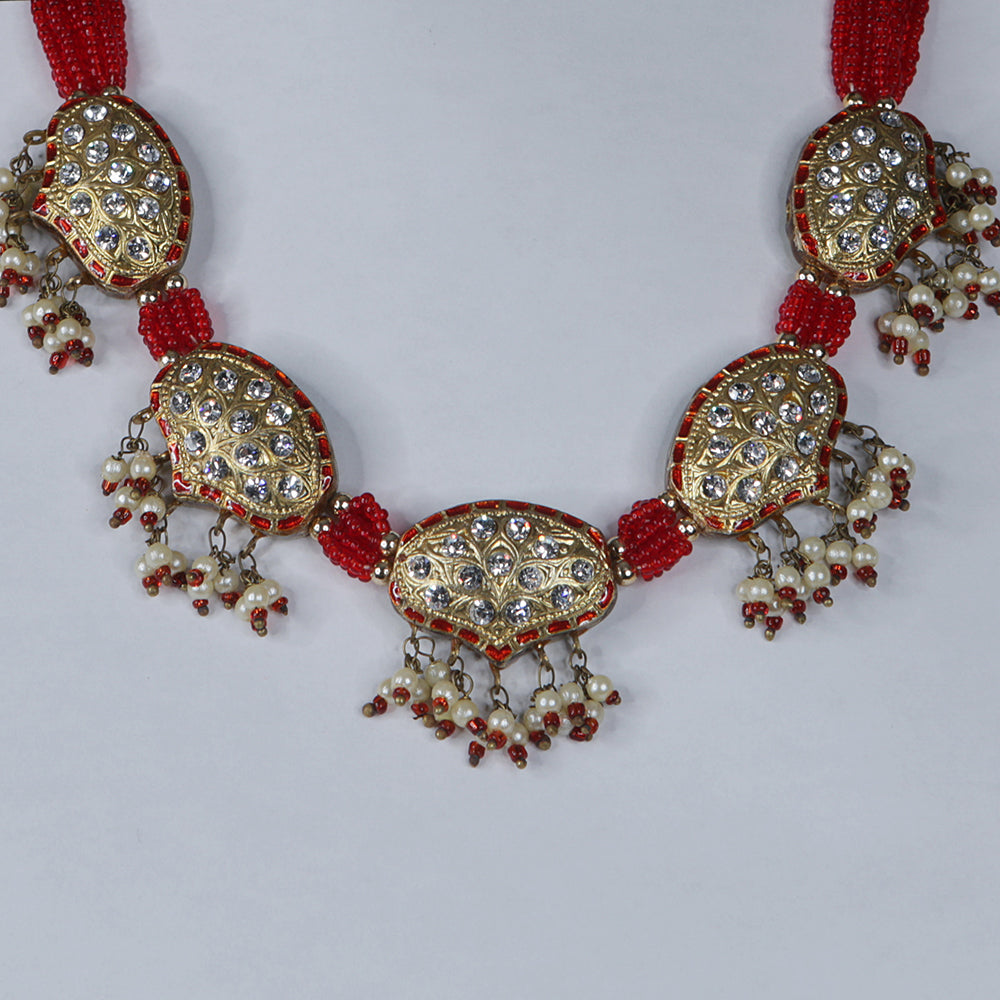The image captures an intricately designed necklace, crafted with an array of colorful and glittering beads. The necklace descends from the upper left of the photo, curves down to the center, and ascends towards the top right. It features a striking band of small red beads connecting multiple ornate oval sections. These ovals are embellished with a variety of gemstones, including red, blue, and white stones that shimmer like diamonds. Hanging from the central oval are strands of pearl-like beads interwoven with red beads, further enhancing the necklace's elegancy. The entire piece is adorned with gold-colored decorations and secured with gold hooks that hold the beads together, all of which is showcased against a light gray background. This luxurious piece epitomizes both craftsmanship and artistic design.